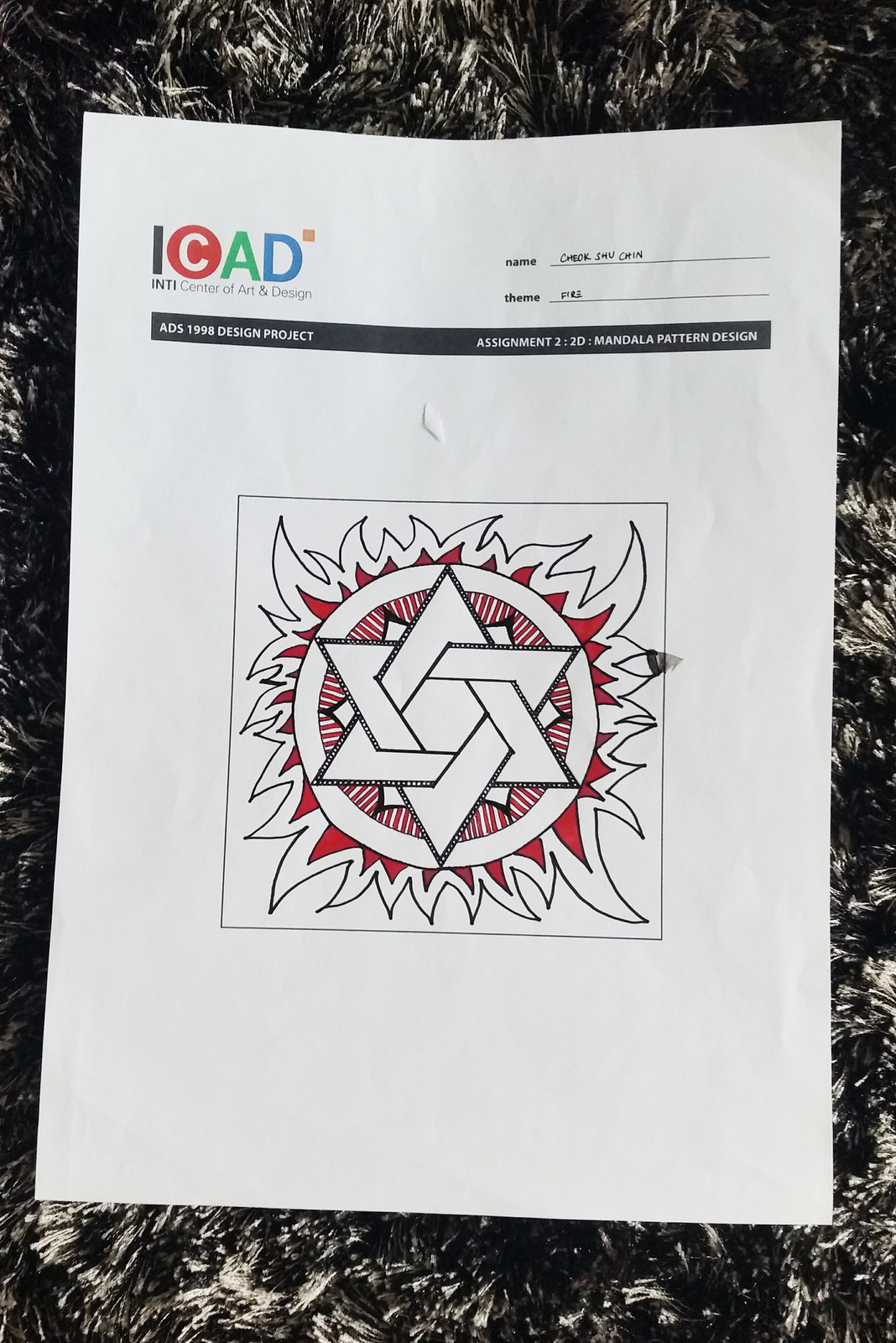This image depicts a printed page resting on a textured, fuzzy blanket. The intricate details of the blanket's fibers are visible, providing a tactile contrast to the smooth surface of the page. 

At the top left corner of the page, there's a logo for "I CAD" featuring the colors red, green, and blue. To the right of the logo, the page has a section labeled "Name" with a line beside it, where a name is handwritten but too small to decipher. Below this, there's another label "Theme" with a line next to it, and something is written there as well, but it's also illegible due to its size. 

A black bar spans the width of the page below these sections, displaying the text "ADS 1998 Design Projects" in white. Following a significant blank space, the text "Assignment 2: 2D Mandala Pattern Design" appears. 

The bottom half of the page features a black-outlined square at its center. Within this square lies a complex mandala design, incorporating flame motifs and geometric patterns. The central design includes interlocking six-sided stars, creating an intricate and symmetric pattern. The mandala is primarily outlined in black, with red accents highlighting the flame-like elements around it. The combination of stark black lines and vibrant red fills gives the mandala a striking appearance.